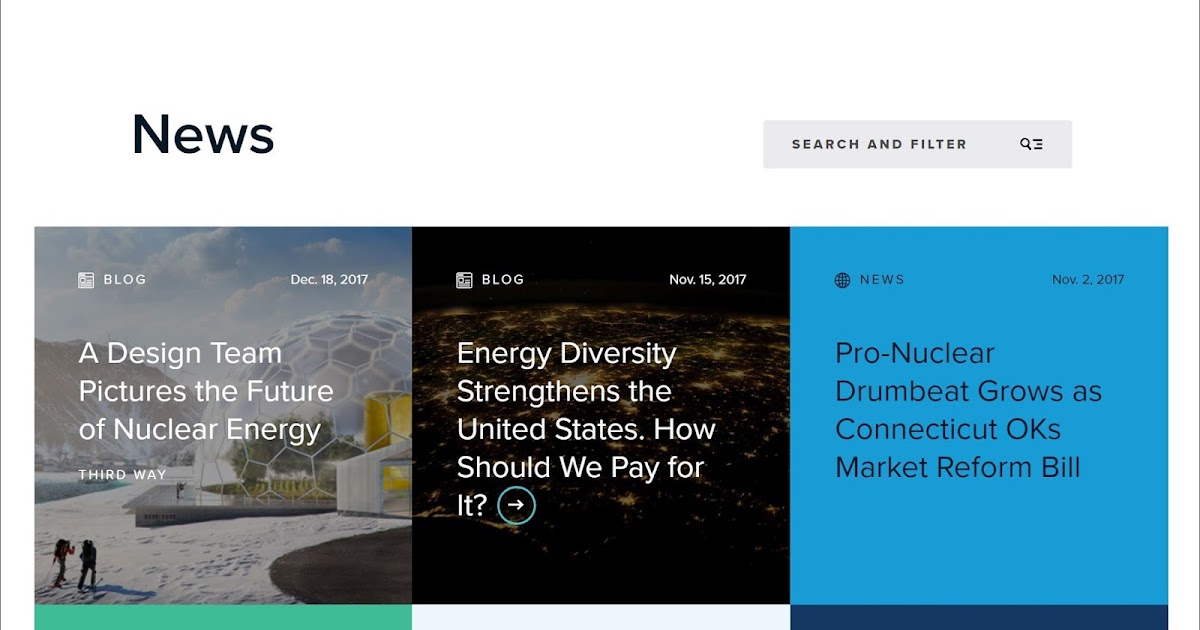In this screenshot of an unidentified news webpage, we see a structured layout that begins with a vertical black line on the left side and another on the right side, framing the content in between.

At the top, the word "News" is prominently displayed in bold black letters. To the right of this heading, there is a search and filter button featuring a magnifying glass icon alongside a menu icon.

Below this header, there are three distinct article boxes lined up horizontally:

1. **The first box**:
    - Label: "Blog"
    - Date: December 18, 2017
    - Title: "Design team pictures the future of nuclear energy"
    - Additional Text: "Third Way"
    - Note: Includes a small, indistinguishable icon or logo next to the "Blog" label.

2. **The second box**:
    - Label: "Blog"
    - Date: November 15, 2017
    - Title: "Energy Diversity strengthens the United States. How should we pay for it?"
    - Additional Feature: An arrow icon, possibly indicating further navigation or action.

3. **The third box**:
    - Label: "News" in a blue square
    - Date: November 2, 2017
    - Title: "Pro-nuclear drumbeat grows as Connecticut OKs market reform bill"

Each of these articles hints at topics related to energy, particularly nuclear energy, and its implications for future developments and policy reforms.